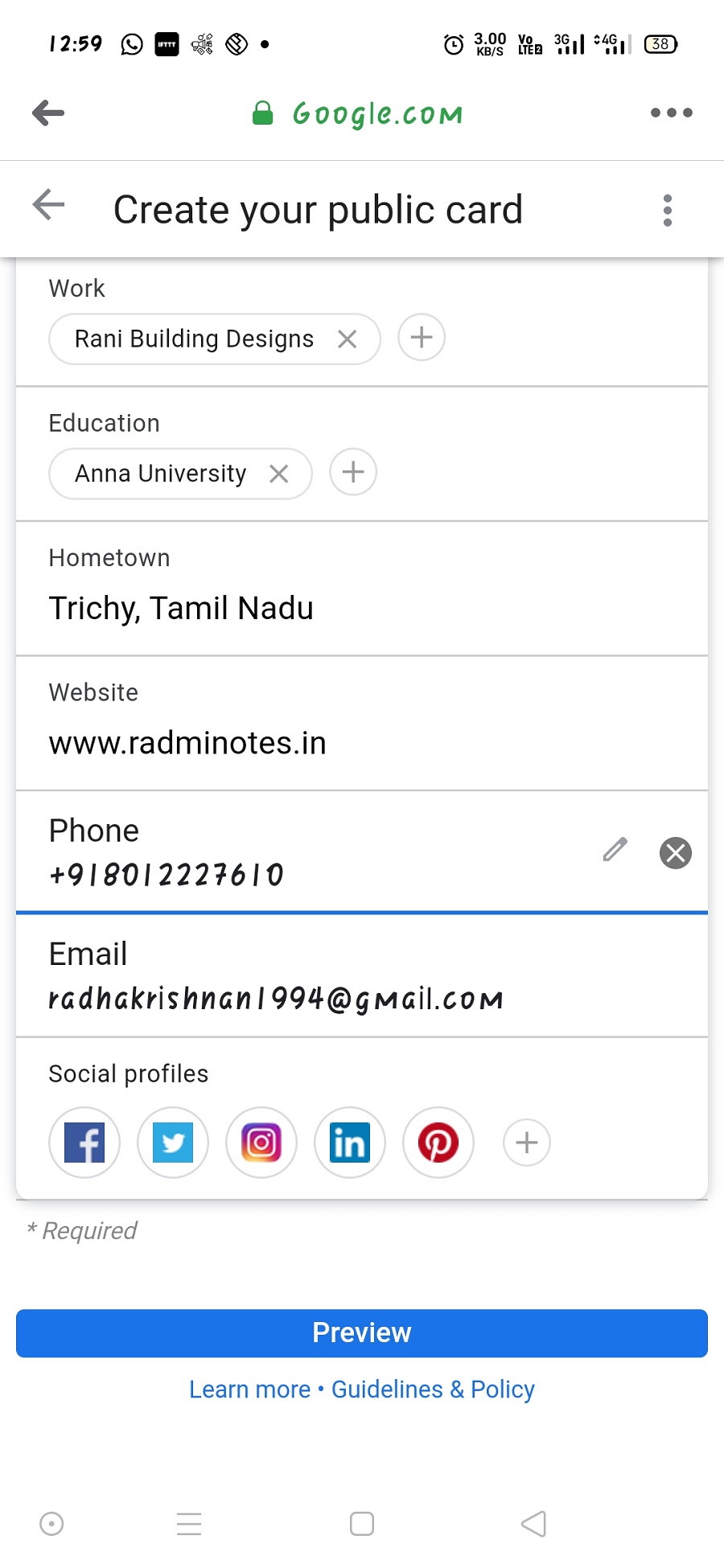The image appears to be a screenshot taken from a smartphone, displaying a Google service page. The page has 'google.com' written in green letters next to a lock symbol, indicating a secure connection. The heading 'Create Your Public Card' is prominent, indicating a step-by-step process for creating a public profile.

In the 'Work' section, the name "Rani Building Designs" is filled in, suggesting it is the user's place of work or business. The 'Education' field lists "Anna University," indicating the user's educational background. The 'Hometown' section is noted as "Trichy, Tamil Nadu," revealing the user's place of origin. A website URL, "www.redminnotes.in," is also provided.

The 'Phone' section lists an international phone number, denoted as being outside the user's home country. The email address displayed is "RADHAKRISHNL994@gmail.com." Social profiles linked to the user include Facebook, Twitter, Instagram, LinkedIn (abbreviated as "In"), and Pinterest.

At the bottom of the page is a statement noting that fields marked with an asterisk are required. A blue button labeled 'Preview' can be clicked to review the public card. Additionally, there is a 'Learn More' link for guidelines and policies, presumably to provide further information about the service.